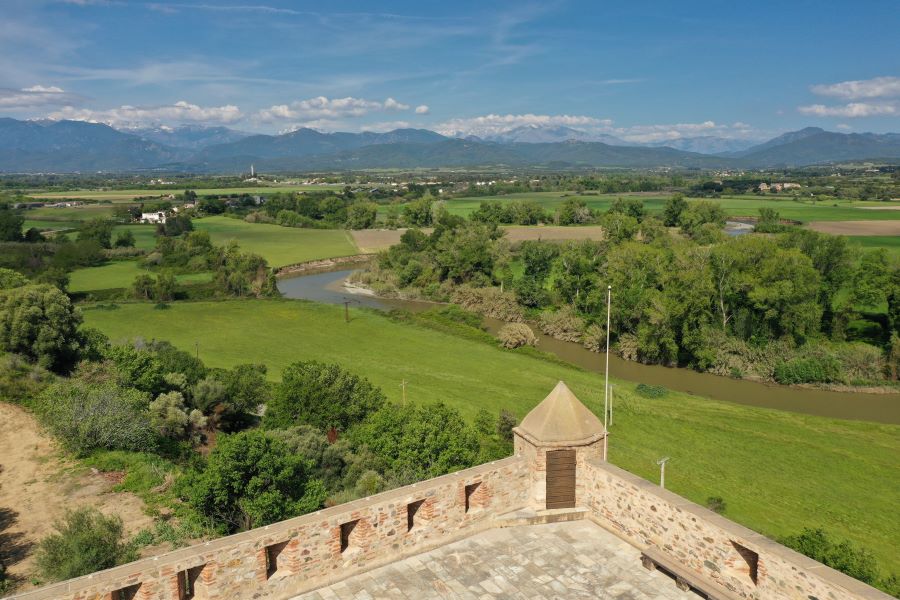This rectangular, wide-angled image beautifully captures a vast outdoor landscape under a bright blue sky with a few clouds hovering near the base of the distant mountain range. The foreground showcases an elegant, castle-like structure made from brick and stone, with a distinctive octagonal corner topped with a pointy, brown roof. The stone floor seamlessly transitions into a small brick railing that frames the structure. This overlooks a sprawling, grassy expanse characterized by sections of light and dark green, reminiscent of a golf course with sandy areas that could be bunkers. A creek meanders through the grass, adding a natural element that complements the surrounding bright green trees and bushes. In the far distance, the outline of a town and other houses can be faintly seen, blending into the hazy mountain backdrop.